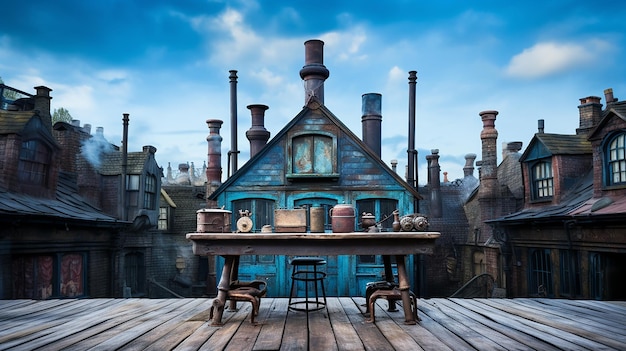This evocative digital image, possibly drawn or computer-generated, appears to channel the aesthetics of a fantasy or steampunk setting, reminiscent of "A Series of Unfortunate Events" or "Willy Wonka." In the foreground, weathered wooden planks form a sprawling deck that stretches across the image. Adorning this deck is a wooden table, accompanied by a stool and a trio of smaller stools tucked beneath. The tabletop is cluttered with an assortment of metal containers and gadgets, including pots and vessels in muted red, gold, and black tones, which hint at intricate, possibly Victorian, steampunk machinery.

Dominating the midground is a quaint blue house made from painted wood, with a prominent chimney jutting from its peak. This house is surrounded by an urban sprawl of closely packed buildings, each topped with a variety of chimneys and smokestacks that differ in styles: some straight with bulges at different points, others slender and more traditional. The chimneys billow with wisps of steam, contributing to the image’s industrial atmosphere. On either side of the blue house, rows of Victorian-style homes, with large windows and towering roofs, continue the theme of a densely-packed cityscape.

Above, a deep blue sky dotted with white clouds frames the scene, adding a touch of serenity to the otherwise bustling and crowded architectural ensemble. Overall, the image paints a detailed and atmospheric portrait of a fantastical, industrial-era cityscape, brimming with intricate details and a rich narrative quality.